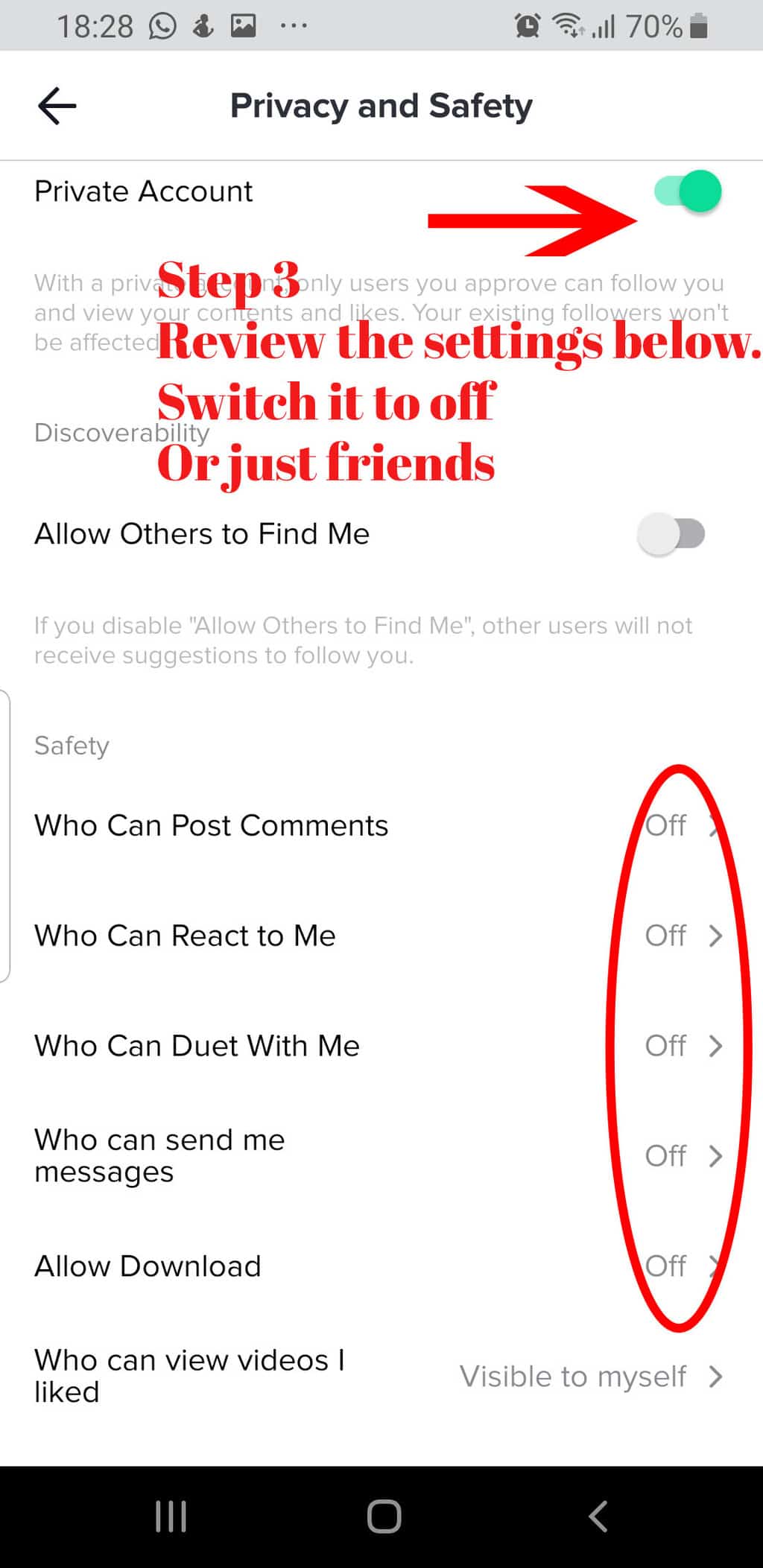A smartphone screen displays a privacy and safety settings page. At the top, within a gray bar, the time is shown as "18:28" on the left, accompanied by various icons including a phone, a running person, and a picture icon. On the right side of the gray bar, the battery level is indicated as 70% along with a battery icon, an alarm icon, and a Wi-Fi icon.

Below the gray bar, on a white section of the screen, the text "Privacy and Safety" is displayed in black, with a back arrow in black pointing to the left. The phrase "Private Account" is written with a red arrow pointing to a green toggle button.

Above this text is a bold, red heading that reads "Step 3: Review the settings below. Switch it to 'Off' or 'Just Friends'." Part of this section is partially obscured by gray text.

The "Allow others to find me" option is displayed as toggled off. Below in the safety section, there are categories each accompanied by right-aligned red ovals stating "Off." The categories include "Who can post comments," "Who can react to me," "Who can duet with me," "Who can send me messages," and "Allow download." Finally, the option "Who can view videos I liked" is marked as "Visible to myself."